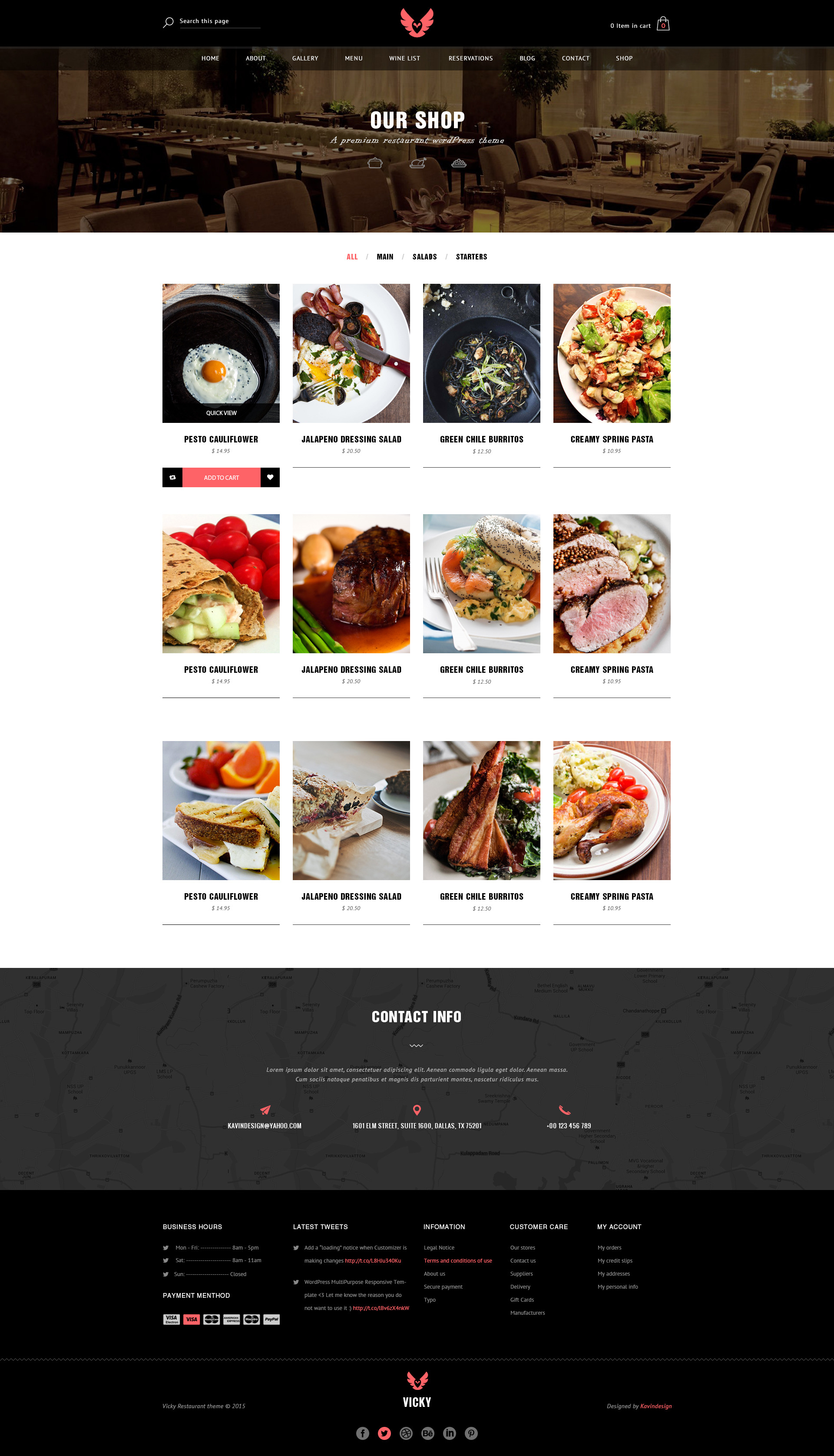A screenshot of a restaurant's website features a dimly lit image of the restaurant's interior, highlighting the seating area at the top. Superimposed on this image is the phrase "Our Shop". The website's main navigation menu is visible above this picture, but the text is too small to be legible. Below the main image, there are 12 small square thumbnail images displaying various food dishes offered by the restaurant. Recognizable dishes include a salad, a steak and egg platter, a wrap, and a sandwich. At the bottom of the page, there is a black bar containing more text, presumed to be options for contacting the restaurant and other relevant information, though the text is also too small to be easily read.